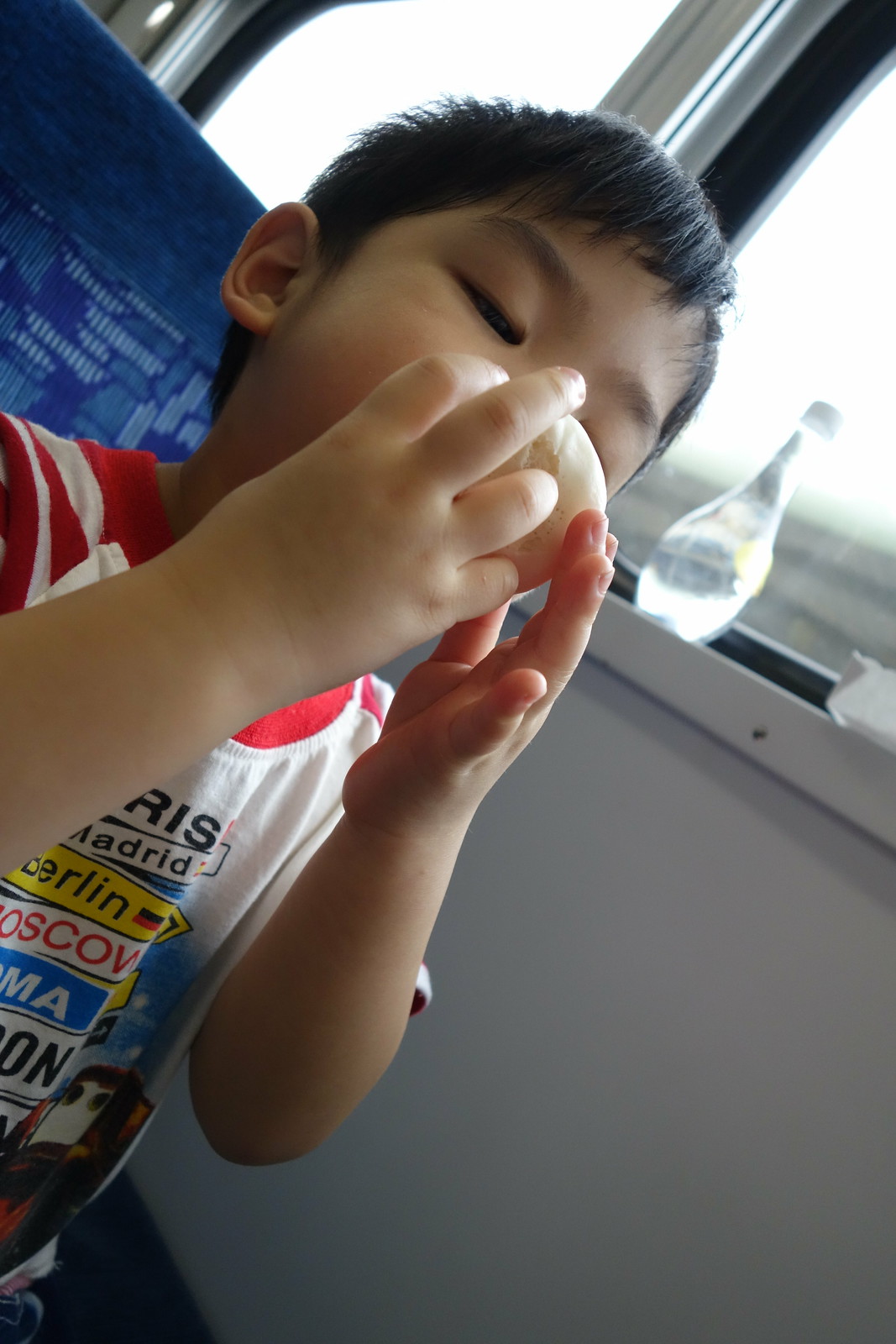In this detailed image, a young boy of Asian descent is depicted sitting on what appears to be a blue train or bus seat. The picture is taken at a slight angle, capturing the scene from his stomach upwards. The boy's short, dark brown to black hair frames his face, where his right eye can be seen looking downward. His hands, holding a white pastry or bread-like food, are raised in front of his face. The boy is wearing a distinctive short-sleeve t-shirt with a red crew neck collar and red accents on the sleeves. The shirt is predominantly white, adorned with various colorful city names such as Madrid, Berlin, and Moscow, pointed out by arrows resembling street signs. The background elements further contextualize the setting: to the right of the boy is a gray wall and a window sill with a white-capped bottle of water. The window behind him provides a glimpse of passing scenery. The scene suggests the boy is captured mid-journey, possibly on a train or bus, enjoying a snack while gazing downward in a casual, candid moment.